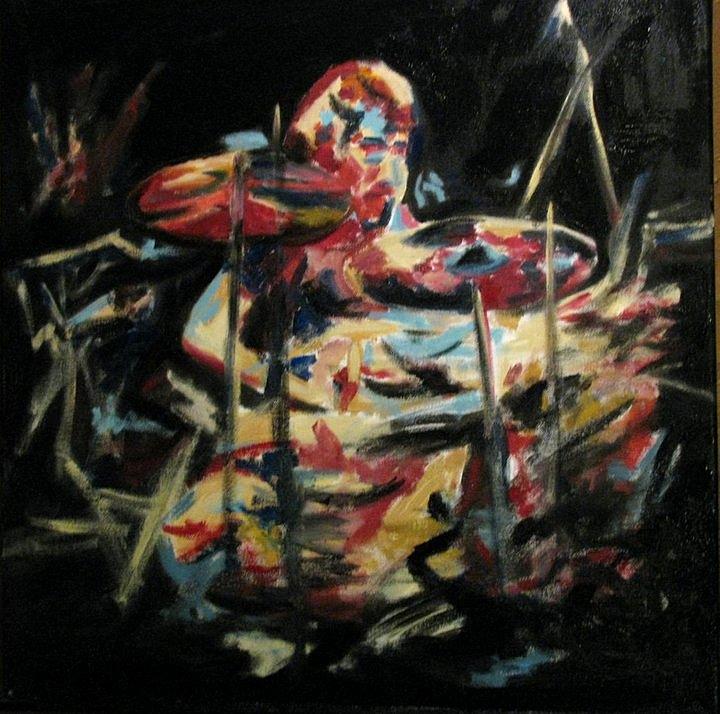The image depicts an abstract painting of a drummer seated at a drum set, set against an entirely black background. The composition is characterized by fluid brush strokes that meld seamlessly to form the shape and outline of the musician and their instrument. You can discern the two cymbals quite clearly, alongside the drum set, and there are suggestions of the drummer’s head and right arm. The painting employs a striking palette of reds, yellows, blues, and occasional blacks to create the visual elements. The colors and brush strokes intermingle in varied directions, contributing to a sense of motion and energy. The drummer appears to be wearing a vibrant outfit with reds, blues, yellows, and blacks, which blend into the surrounding abstract elements, enhancing the overall dynamic feel of the piece.